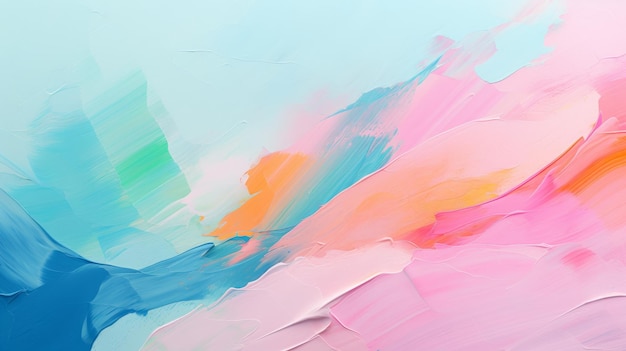The image showcases an abstract acrylic painting characterized by a gradient of colors, including blues, pinks, pastel greens, and hints of orange and purple. The canvas is adorned with broad brush strokes, creating a layered effect, indicative of the artist’s technique. The use of a scabble or a spoon is evident in the textured shapes and smears. Starting from the top left, the painting features baby blue transitioning into teal, while the bottom left corner has a dark blue smeared into light blue. Moving right, baby blue mingles with a touch of orange, and light pink is introduced. The central area blends blues and oranges, leading to the right half dominated by various shades of pink, from baby pink to darker pinks, with sporadic streaks of orange and purple adding complexity. The overall effect is a rich, textured portrayal of colors melding seamlessly into one another.